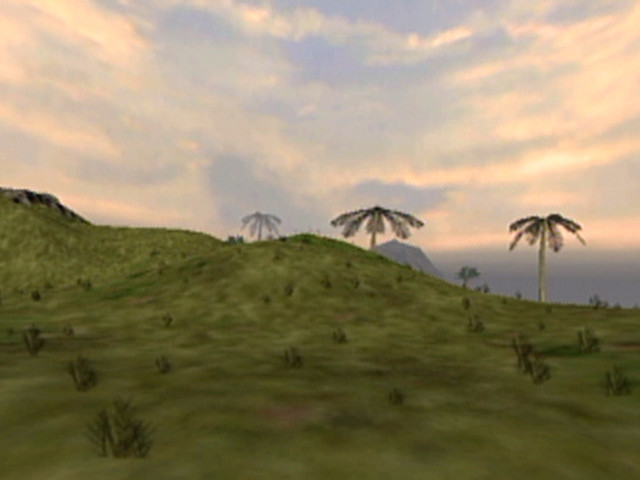This intricate digital artwork, reminiscent of a Jurassic landscape or a video game scene, depicts a vast, green field stretching from the middle of the image to the corners. The terrain features gentle hills and inclines, with the lush green grass dotted by small, dark green bushes or cacti. Notable in the foreground and midground are several tall palm trees with unusual, downward-aimed fronds. You can spot one prominently on top of a hill, another to the right, and a few more off in the distance, creating a layered effect. Adding to the varied landscape, some hillsides also showcase rocky outcrops. In the far background, a distinct mountain or large hill rises, its peak barely visible. The sky above is a tapestry of light blue and gray hues with numerous white clouds, suggesting a very cloudy day, although some sunlight pierces through, notably brightening the right-hand side of the image. The overall ambiance hints at dusk, with the interplay of light and shadow adding a dramatic touch to this vast, prehistoric-like scenery.